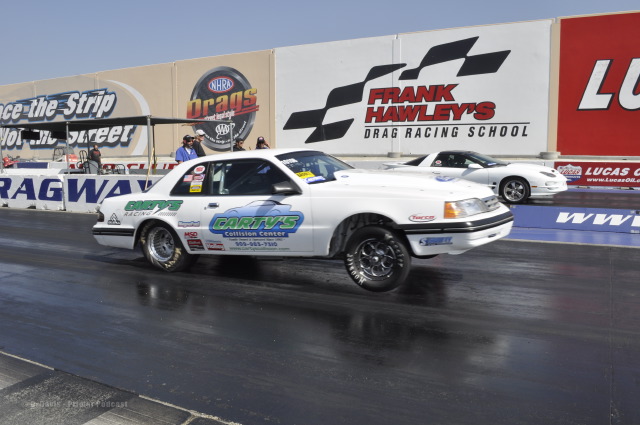The image depicts an exhilarating moment on a sunlit drag strip, with two cars racing against each other. In the foreground, there is a classic white coupe with its front tires lifted off the ground, marked with "Cartes Collision Center" on its door in green letters on a blue background. This car, possibly a vintage Ford, has darkly tinted windows. Right behind it is another white car, equally poised for the race. Both cars are separated by a center divider, around which several people are gathered, standing under a cover. The black pavement stretches beneath the cars as they speed along.

The background features a tan wall adorned with numerous racing-related signs and logos, most prominently "Frank Hawley's Drag Racing School" in red and black letters, complemented by a checkered racing flag. Other visible signs include “NHRA” in white on a blue background, “Braggs” in vibrant orange and red, the “AAA” symbol in white on black, and parts of a "Lucas" sign in white on red. The wall beside the divider also carries the words “Bragg Way” in blue letters on a white background. The entire scene exudes the high-octane atmosphere of a competitive drag racing event, capturing the essence of speed and excitement.